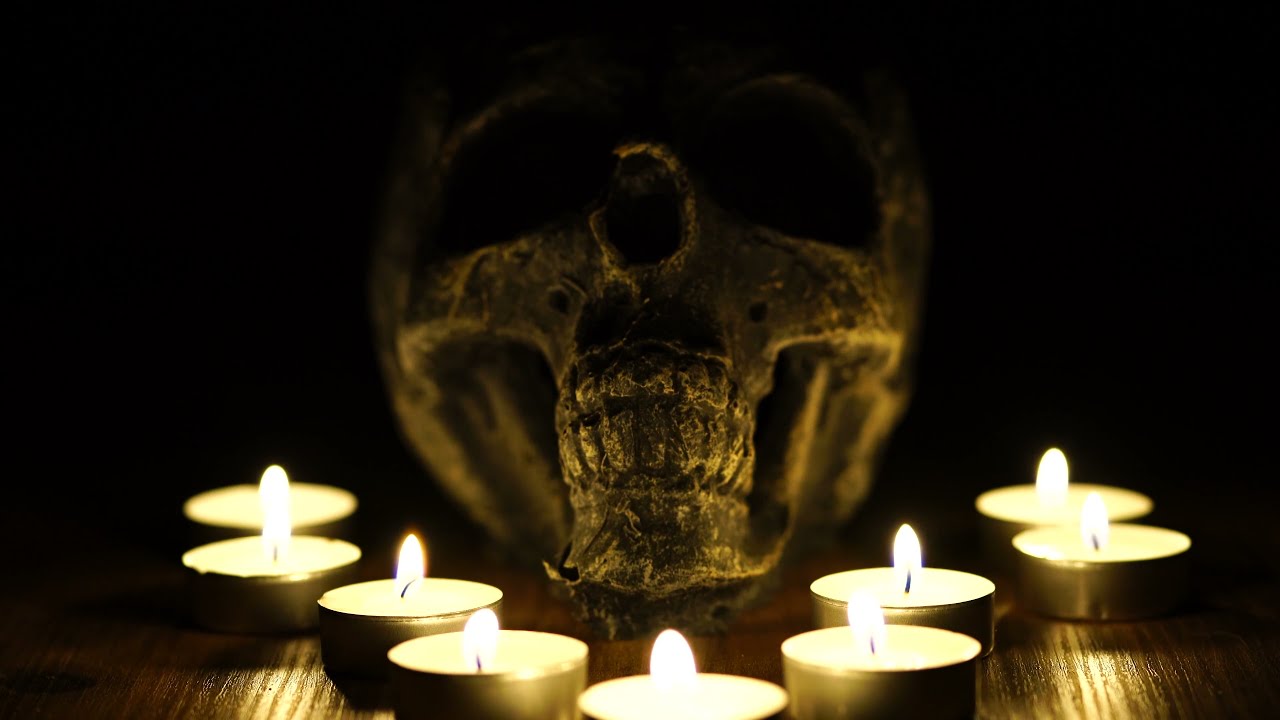This eerie image depicts an ominous scene set in an extremely dark room with only the faint, flickering light of lit tea candles to illuminate it. At the center, taking up most of the frame, is a large, decomposing human-like skull, positioned on a wooden table. Its disfigured nose and absent cheekbones add to its unsettling appearance, while the large eye sockets and narrow, fused-together teeth suggest it may be a statue rather than a real skull, possibly made of bronze or metal. The candles, arranged in a V-shape with four on each side and one at the point, cast a yellowish hue onto the skull, further enhancing the macabre and grim atmosphere. This chilling setup, with its dark, black background and sinister focal point, could be interpreted as something related to sacrificial rituals or Halloween decorations.